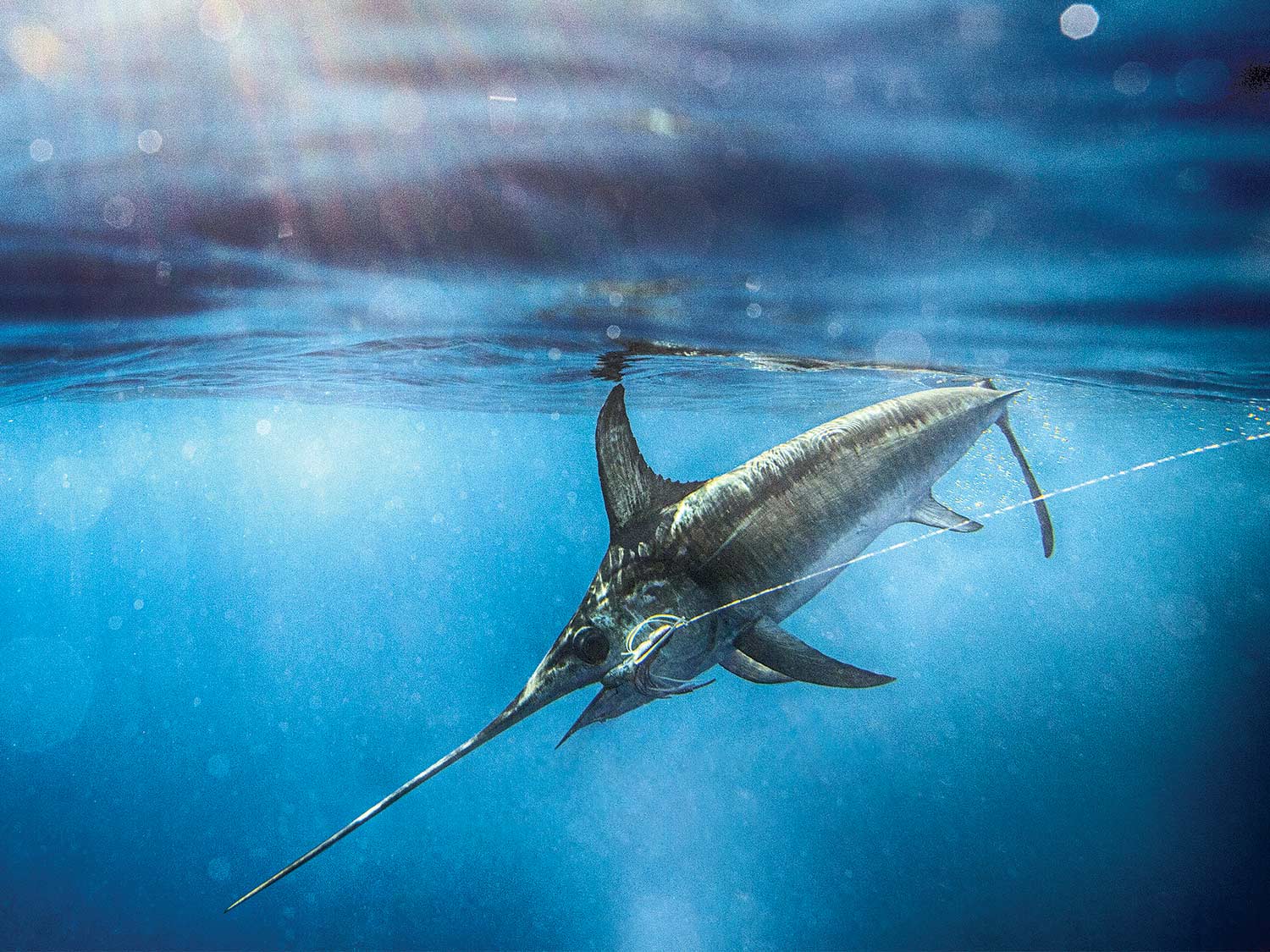This is a detailed, horizontally aligned, full-color underwater photograph captured during the daytime. The clear, very blue water is illuminated by sunlight streaming through, creating diagonal vertical rays and a backdrop of bubbles. Just below the ocean's surface, a medium-sized swordfish is seen in motion, identifiable by its long, pointed snout or "horn," which protrudes out sharply. The fish’s mouth is open, revealing it to be mostly gray with a silvery hue, accented by white or silver spots around its face and a prominent large black eye. Positioned towards the left, the swordfish appears caught, with a fishing lure and hook visible on the side of its face. This lure trails a fishing line that leads up towards the upper right corner of the image. The background features a gradient of light blue mixed with white, with the top part appearing extra blurry, highlighting the dynamic, natural setting of this underwater scene.